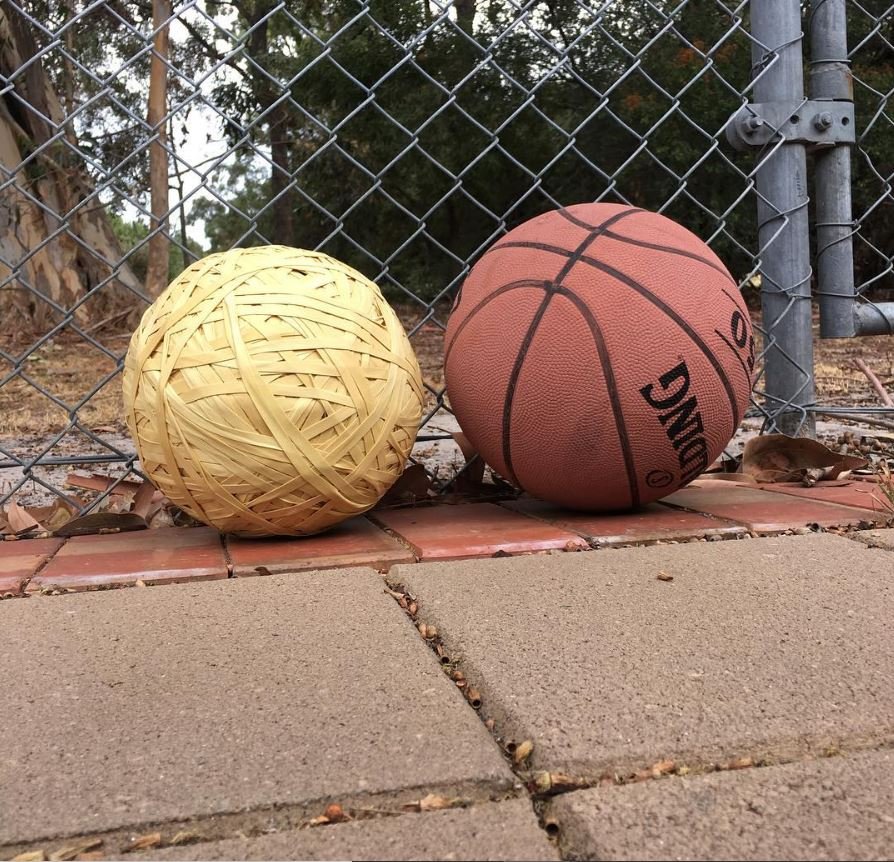The image depicts an outdoor park or playground area, likely in an urban setting, characterized by a mix of concrete tiles and red brick rows. Dominating the center of the image are two notable objects: an orange basketball labeled "Spalding" in black, and a similarly-sized, tan rubber band ball. Both balls rest on the red brick section, leaning against a metal chain-link fence. The gray, square concrete tiles form the foreground, while the background reveals a somewhat unkempt, forested area with visible trees, patches of sky, and scattered leaves, suggesting it is autumn. The setting appears to be documented during the daytime.